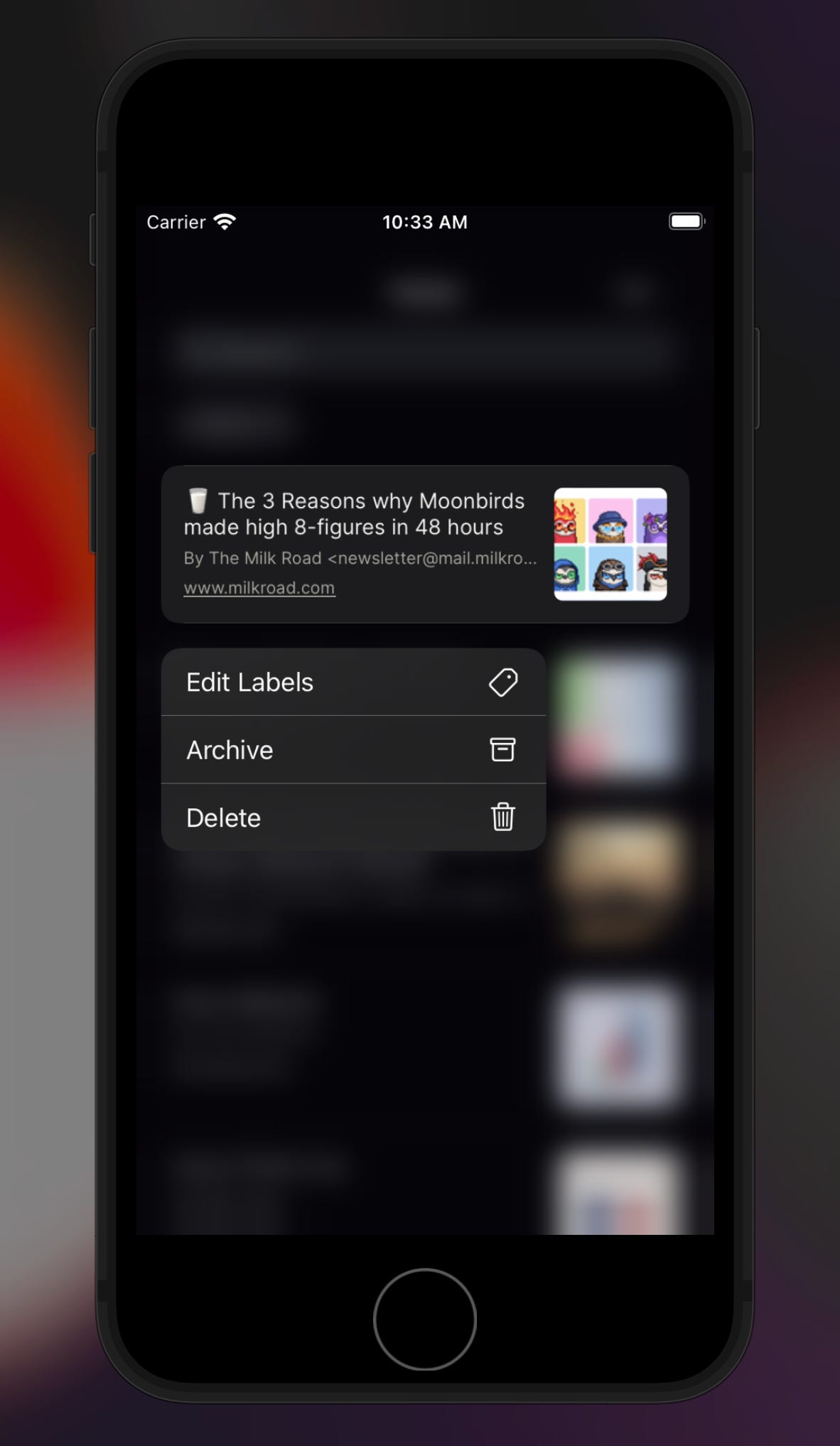The image is a rectangular photograph with a dark, out-of-focus background dominated by shades of black and dark gray. At the center of the composition is a close-up shot of a smartphone screen. 

In the upper left corner of the phone screen, "Carrier" is displayed along with a wireless signal icon. Centered at the top is the time, "10:33 AM," while the upper right corner features an almost full battery icon.

The main content on the screen consists of white text against a dark gray background, which reads: "The top three reasons why Moon birds made high eight figures in 48 hours by The Milk Road. Newsletter at mail dot milk roo dot dot dot. www.milkroad.com." Adjacent to this text, on the right-hand side, is a thumbnail icon displaying several animated characters resembling colorful owls or birds.

Below this section, the words "Edit Labels" appear alongside an icon resembling a price tag on the far right. The next line reads "Archive," accompanied by a file box icon to its right. Further down, the word "Delete" is displayed next to a trash can icon on the far right side.

At the bottom of the phone, the iconic round home button typical of older iPhone models is visible.

The website www.milkroad.com is mentioned twice within the textual content on the screen.